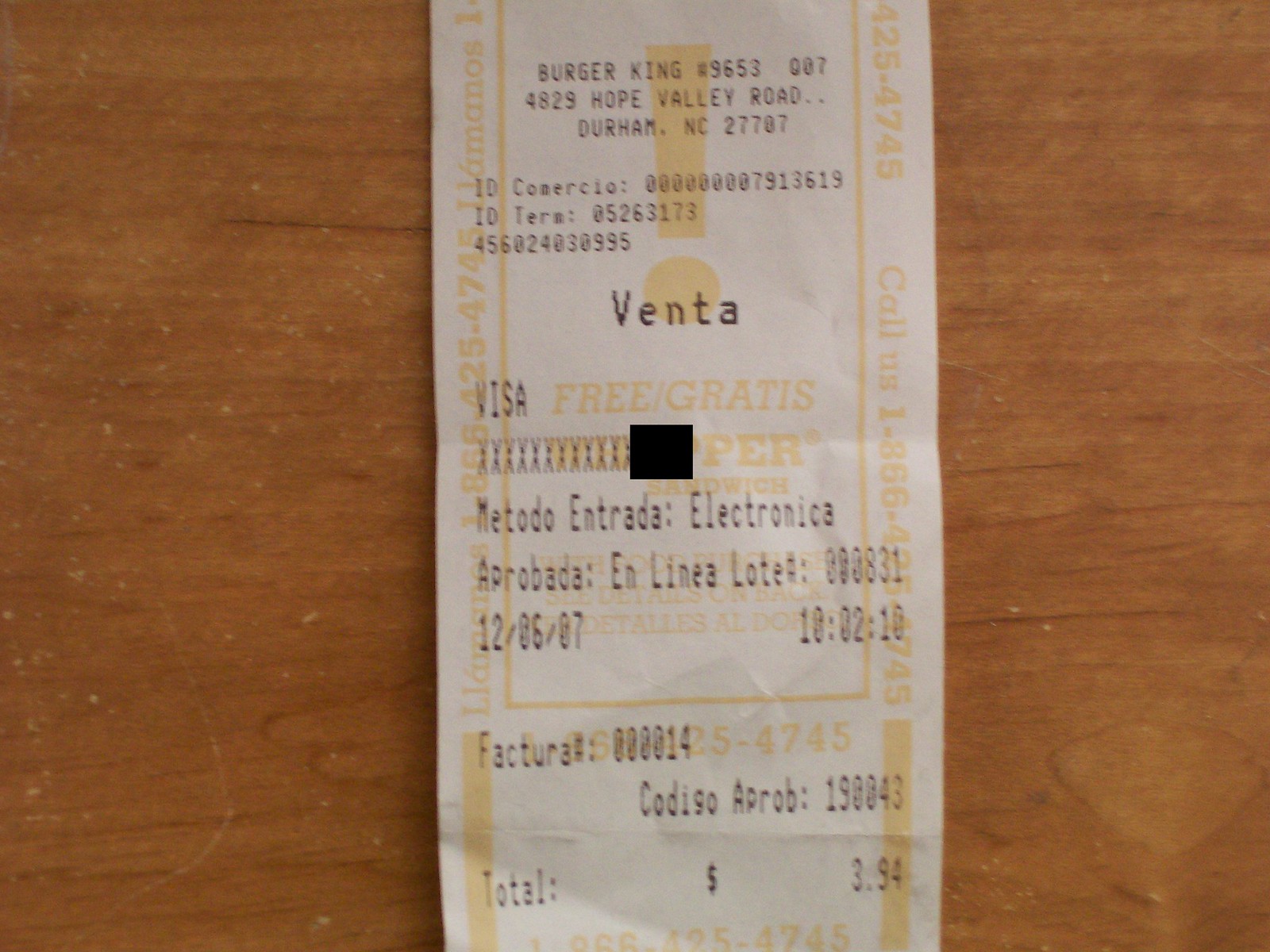This is a color photograph of a white Burger King receipt from 4829 Hope Valley Road, Durham, North Carolina, lying on a golden wooden tabletop with visible grain and some small white flecks and scratches. The receipt features black printing and a yellow Burger King logo in the background. At the top, it reads "Burger King" followed by the location and store number, "59-653-007." Below the store details, it includes terms like "Venta" and "Metodo Entrada Electronica," indicating transactions, with the Visa card information partially blacked out. The receipt is for a purchase made on 12-06-07 at 10:02:16 AM, totaling $3.94. Additional information on the receipt includes transaction ID and approval codes, with some parts of the text in Spanish, such as "Gratis," "Factura," and "Codigo."